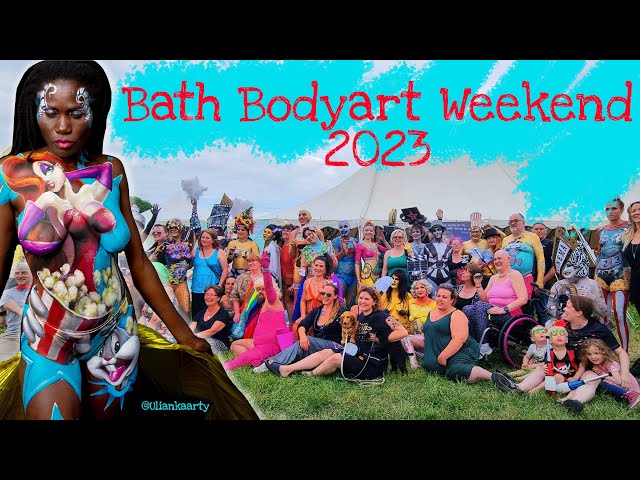The image showcases a promotional flyer for the "Bath Body Art Weekend 2023" event. The flyer is in landscape orientation, framed by black bars at the top and bottom. Across the top, red text reads "Bath Body Art Weekend" on one line and "2023" on the next, set against a speckled blue-teal background. The central part of the flyer features a diverse group of people sitting and standing in an open field, all adorned in vibrant body paint designs rather than traditional clothing. Among the attendees are a person with a dog, another in a wheelchair, and someone resembling the Statue of Liberty.

Prominently positioned on the left-hand side is a larger, transposed image of a black woman with long black hair, entirely covered in body paint. Her face is decorated with white designs, while her upper body and midsection display images of Jessica Rabbit and Bugs Bunny. Notably, Bugs Bunny appears on her left thigh, and a bucket of popcorn being held by Bugs Bunny is painted across her midsection. The crowd, seemingly engrossed in something off to the left, contributes to the dynamic, festive atmosphere of the event.